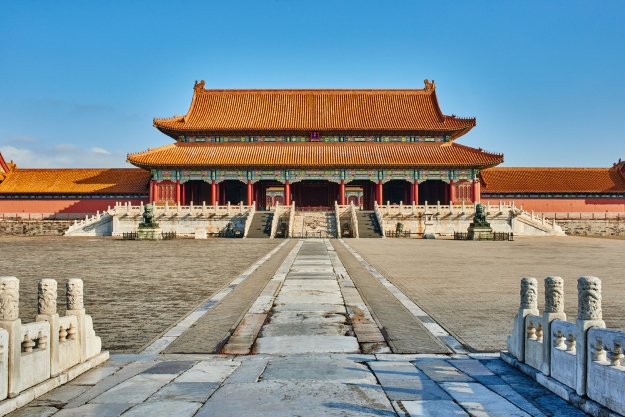This image features an expansive view of the Palace Museum located in the Forbidden City of Beijing, China. The photograph captures the grand building from a distance, allowing a full view of its intricate design. The architecture is highlighted by its traditional Chinese elements, including a distinct brown double roof and green overhanging panels supported by red beams. The structure is adorned with eight arched doorways and a central main archway, creating a sense of symmetry and grandeur.

Leading up to the building are stone pathways and ceremonial bridge-like structures, flanked by sculpted concrete poles at the front corners of the image. The scene is illuminated by clear blue skies and bright sunlight, emphasizing the vibrant colors of the building’s red, white, and orange-ish hues. Flanking the entrance, there are possible statues, potentially depicting foo dogs, although they appear distant and slightly indistinct.

The empty grounds and absence of people suggest this photo was taken before the museum opens to the public, providing an uninterrupted view of the majestic architecture and stone walkways.